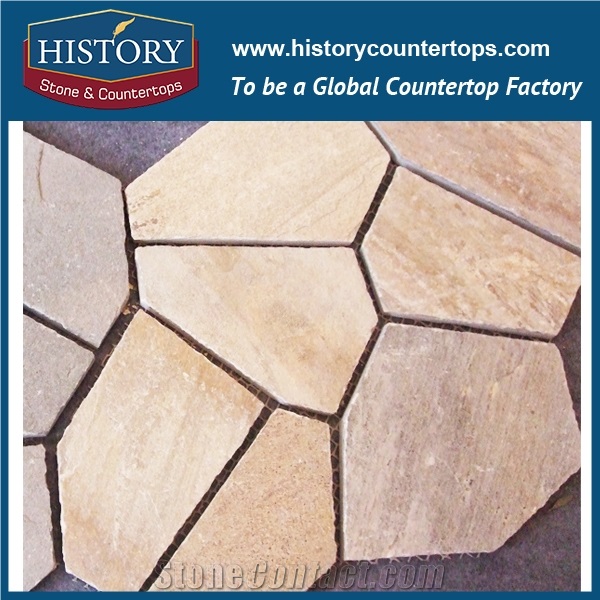The image displays a reklama promoting a countertop company. Dominated by a square banner, the advertisement features a thick border at the top and thin borders on the sides and bottom. At the center of the image is a visually engaging geometric design composed of interlocking, flat stone pieces in hues ranging from light brown to pinkish brown, set against a dark gray rock background.

At the top, a medium blue banner spans from left to right, bearing the text "History" in white within a box. A feather sticks out of the 'T', adding a unique logo detail encased in a hexagonal gold border. Below it, a red banner with white text reads "Stone and Countertops." Further information follows in another line of white text on the blue background, indicating the website "www.historycountertops.com" and the company’s ambition "To be a global countertop factory." The cohesive layout and precise detailing present a professional and polished look, effectively showcasing the company's product and branding.